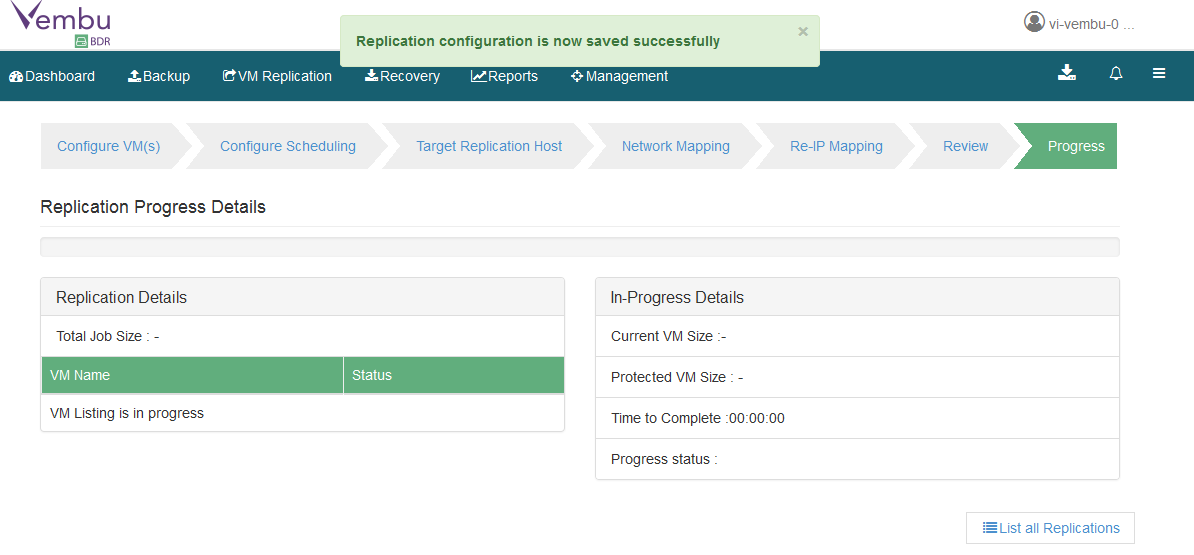Here is a detailed and cleaned-up caption for the provided image description:

---

This web page appears to be part of the VEM VEU application interface, featuring a predominantly white background. 

**Top Section:**
- In the top left corner, "VEM VEU" is written in purple, accompanied by smaller, indistinguishable text also in purple and a small green square to its left.
- At the top of the page, there is a light green notification bar reading "Replication configuration is now saved successfully" in darker green, with a gray "X" on the upper right-hand corner to dismiss it.
- An idealized profile picture appears on the far right of the notification bar, next to unreadable gray text.

**Navigation Bar:**
- Directly below, a darker, bluish-green horizontal navigation bar spans the width of the page.
  - On the left, it starts with a "Dashboard" icon and text in white.
  - Next, a person-shaped icon labeled "Backup" in white.
  - Followed by an icon labeled "VEM Replication" in white.
  - A download icon labeled "Recovery" in white.
  - A checkmark in a box labeled "Reports" in white.
  - Another indistinguishable icon next to "Management" in white.
  - On the far right, this bar includes a download icon, a bell icon, and a three-bars icon, all in white.

**Content Area:**
- Below the navigation bar, the page features a series of gray horizontal boxes with arrows pointing to sections labeled in dark blue:
  1. Contiguous VMs
  2. Continuous Scheduling
  3. Target Replication Host
  4. Network Mapping
  5. RE-IP Mapping
  6. Review
  7. A darker green box labeled "Progress" in white.

**Replication Details Section:**
- Below these, the section labeled "Replication Progress Details" in black precedes a thin gray line spanning the page's width, followed by a thicker gray line.
- The text "Replication Details" appears in black over another gray line extending halfway across the page.
- Underneath is a white section stating "Total Job Size" in black, and a green area labeled "VM Name" in white, followed by small white bars marked "Status".
- Halfway down, another white bar states, "VM Listing in Progress" in tiny black print, filling half the page width.

**Progress Details Section:**
- To the right, a gray bar reads "In Progress Details" in black.
- Below are several white-text sections:
  1. Current VM Size in black.
  2. Protected VM Size in black.
  3. Time to Complete (showing 00:00:00).
  4. Progress Status in black.

**Bottom Section:**
- At the very bottom right, "List All Replications" is shown in blue, with small blue bars to its left.

---

This detailed and formatted description outlines the web page's major elements and their positions, providing a comprehensive overview of the interface.